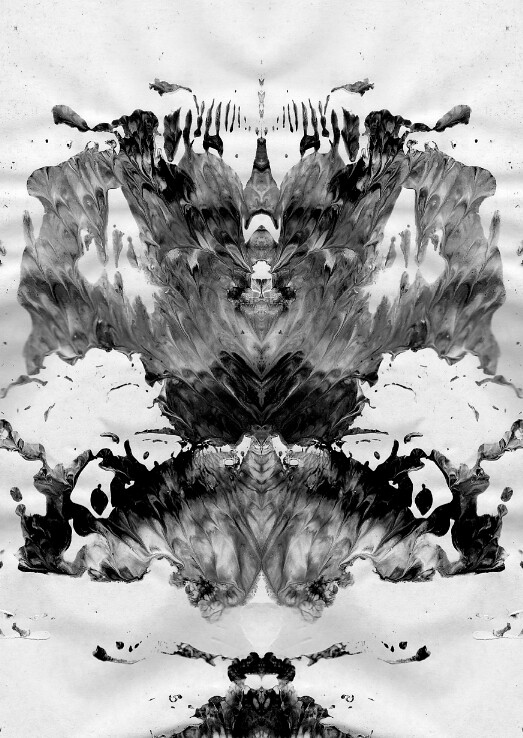This black and white abstract artwork, resembling an intricate inkblot test, showcases a rich array of symmetrical designs and shapes. The rectangular, vertically-oriented piece employs a combination of light and dark shades to create a dynamic visual journey from bottom to top. The base of the image is reminiscent of snow, leading up to striking patterns that resemble the mirror-imaged faces of dogs with noticeable eyes and noses. Dividing these canine figures is a central, monstrous form. Above this area, a shape reminiscent of a cotton ball transitions further upwards into what appears to be bats with wings, adding to the layered complexity of the artwork. The very middle of the piece features shapes that suggest a bottle, while the top is adorned with various splotches indicative of a diverse, almost celestial sky.